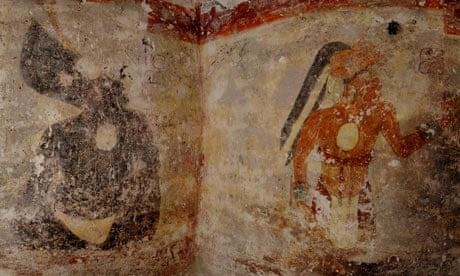The image depicts an ancient cave painting on the side of a stone wall, characterized by its age and weathered appearance. The surface of the wall exhibits a variety of colors including white, brown, and red hues, creating a rough, textured backdrop. On the left side of the painting, there is a black figure, ambiguously resembling either a seated man blowing a trumpet or simply abstract markings. The right side showcases a dark-skinned figure, identified as a warrior or man, possibly from the Aztec civilization. This figure strikes a dynamic pose with arms positioned as if preparing to run. He sports a traditional headdress with long black and white strands extending down, possibly to his elbow, and wears a prominent, circular necklace that could potentially be a large, flat shell. An orange-brown line, resembling fencing, runs across the top of the painting, adding to the overall depth and detail of the ancient artwork.